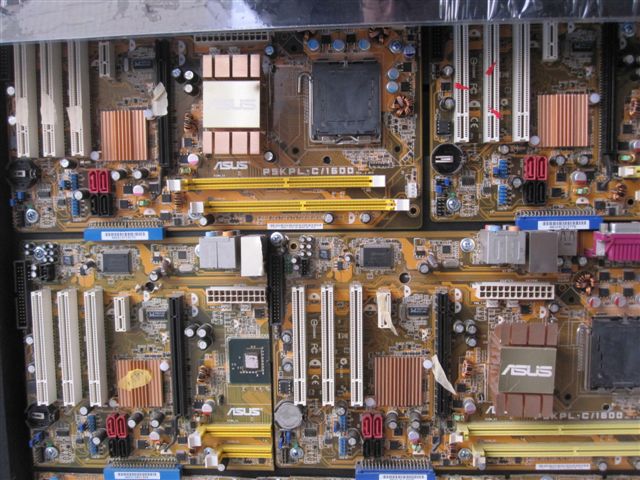The image showcases the interior of what appears to be a computer or a related setup, focusing on multiple ASUS motherboards stacked together. These motherboards feature various empty compartments where additional components like memory and processors would typically be inserted. The boards are branded with multiple ASUS logos, with some textual identifiers such as "PSK, PL, C, slash, 1500". The setup includes several detailed elements: intricate circuits, heat sinks, and a variety of connectors. Three long silver structures and two horizontal yellow components add complexity, resembling a mix of tubes and additional motherboard features. The scene suggests a display setup or a case where these motherboards are showcased, given the visible metal bar at the top of the frame and the absence of active components like fans or processors.